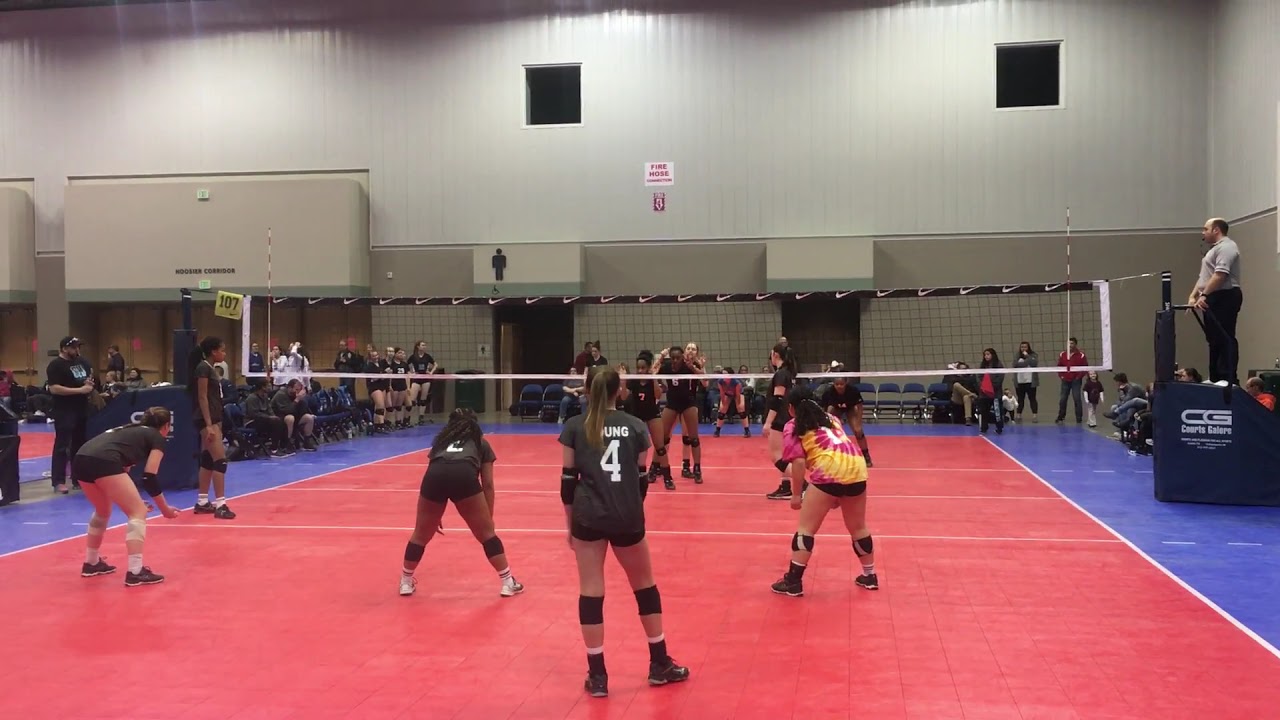This indoor photograph captures an intense volleyball match between two all-female teams in a well-lit gymnasium with white upper and light gray lower walls. The court surface is predominantly red, bordered by a royal blue outline, and features interconnected puzzle-style mats. A highly focused referee stands poised on the right, atop a stand decorated with a CG logo and nike swooshes emblazoned across the black net that divides the teams. Players are deeply engaged, attired mainly in black shorts, knee pads, and shoes, some sporting numbers and names on their jerseys. A girl on the near right side of the court stands out in a magenta and yellow tie-dye shirt. In the backdrop, sparse spectators are seated in blue seats, including sections on the left side of the image. Visible are restroom signs marking the men's on the center left, while the women's is implied nearby, suggesting the amenities accessible in this organized indoor competition.